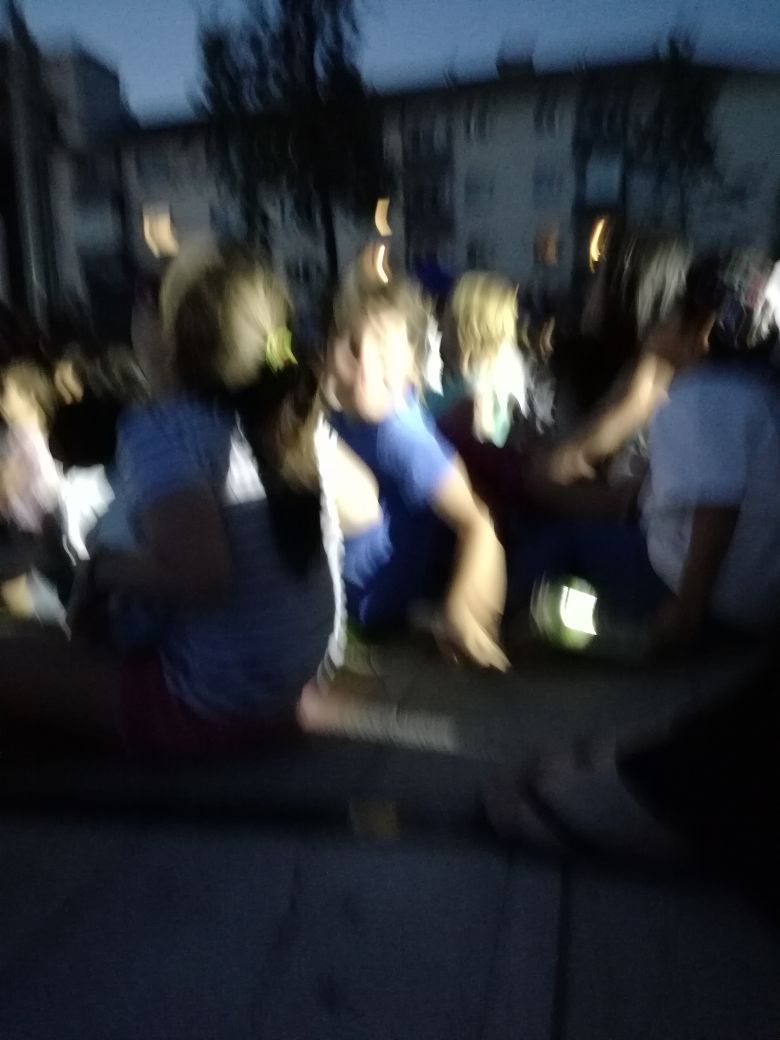A blurry photograph captures a bustling outdoor scene near sunset. In the foreground, two individuals, difficult to identify by gender due to the image's lack of clarity, are dressed in blue clothing. Among the crowd, a person with blonde hair stands out. The background reveals several apartment buildings, silhouetted against the twilight sky which is transitioning from gray to dark. A lone tree is also present in the backdrop, adding a touch of nature to the urban setting. Despite the image's blurriness, it vividly conveys the presence of numerous people enjoying the outdoor atmosphere as daylight fades away.